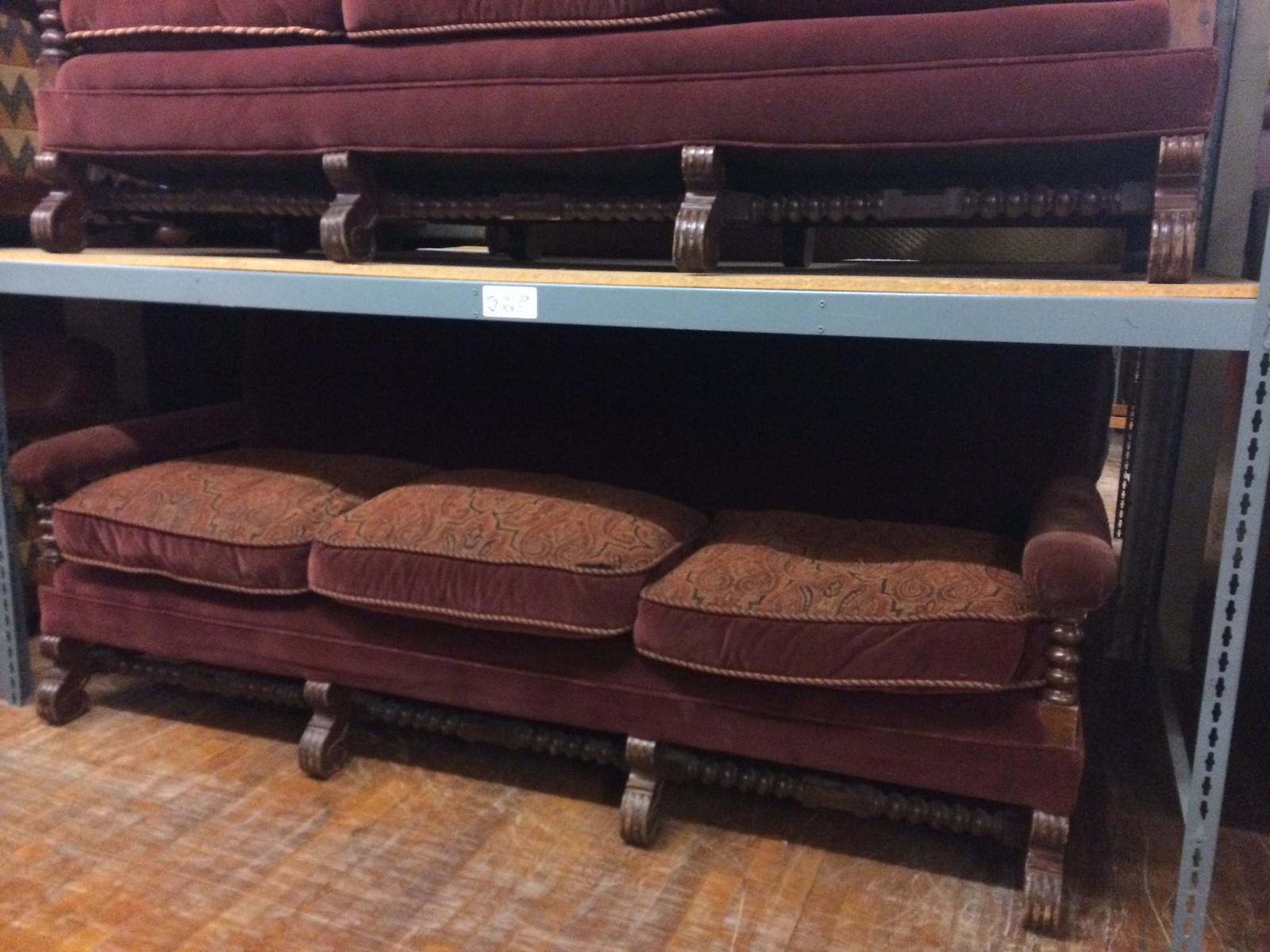This image captures an indoor scene, presumably inside a furniture store. The store's floor is brown and heavily worn with visible scratch marks. Central to the photograph, we see a setup of metal shelving with two similarly designed, ornately decorated couches. The lower couch, positioned on the ground, features reddish-brown cushions with intricate embroidery and is supported by a sturdy wooden frame with four wooden legs. Above it, on a metal shelf, rests another couch of a slightly lighter tone with similar embroidery, further accentuating its antique appearance. The upper couch’s design is primarily visible from the bottoms of its cushions due to its elevated position. Both couches share a robust construction with thick bars connecting their wooden legs. In the background, partially visible, are additional sections of the shelving filled with more furniture. The environment suggests a rustic and varied display designed to showcase the detailed craftsmanship and intricate upholstery of the vintage-style couches.